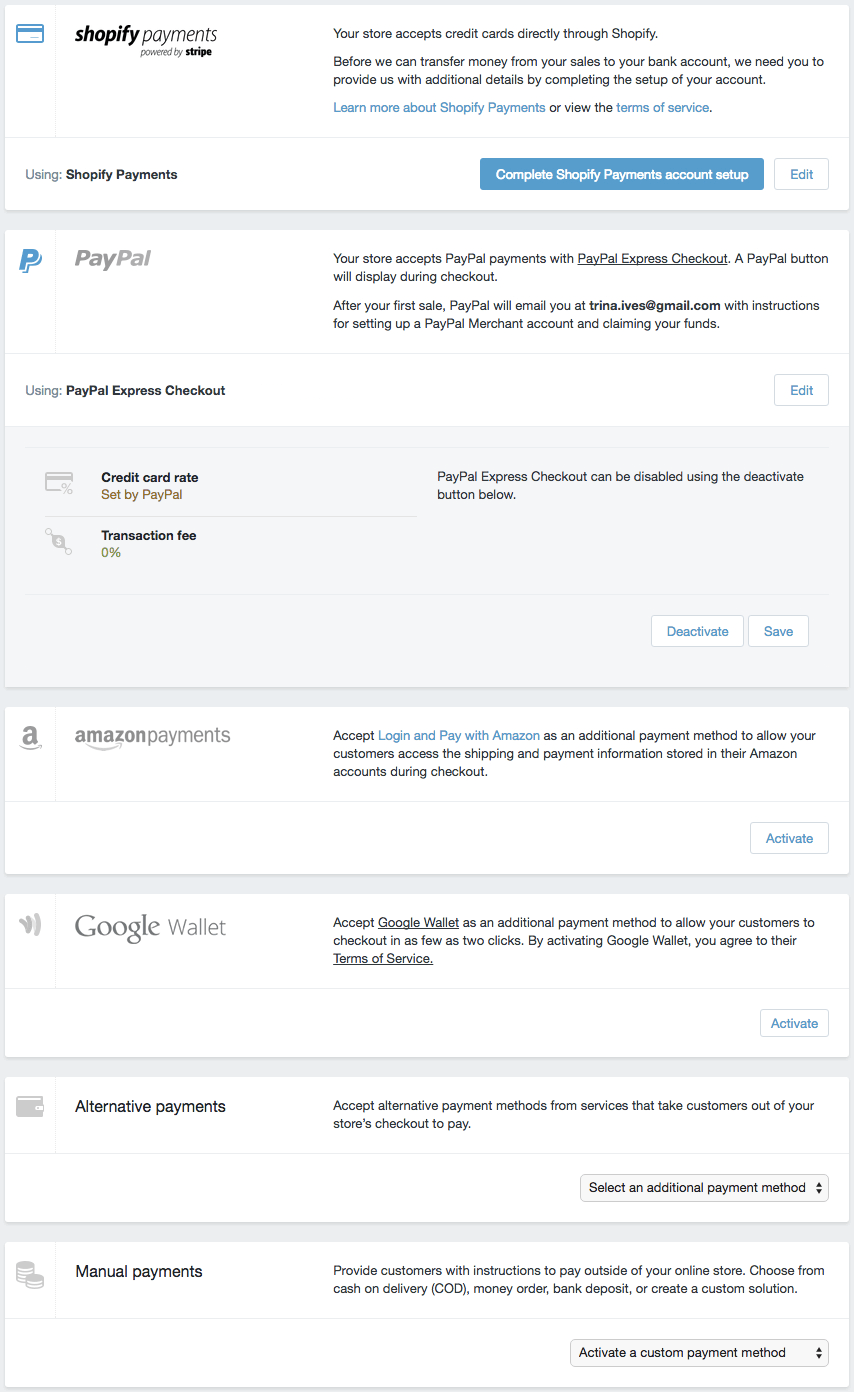The image depicts various Shopify payment options to personalize your store's payment settings.

At the top, there is a section titled "Shopify Payments Powered by Stripe." This section informs that your store can accept credit card payments directly through Shopify. However, to initiate transfers from your sales to your bank account, you need to complete the account setup by providing additional details. There's also a link to learn more about Shopify payments or review the new terms and conditions. Below this information, there's a prominent blue button labeled "Complete Shopify Payment Account Setup" and another button labeled "Edit."

Below this, there's a section about PayPal. It states that your store accepts PayPal payments using PayPal Express Checkout. A PayPal button will appear during the checkout process. Once you make your first PayPal sale, you'll receive an email at trinet.evesgmail.com with instructions for setting up a PayPal Merchant account and claiming your funds. There is a reference to the 0% transaction fee for using PayPal Express Checkout. Additionally, there is an "Activate or Save" button for enabling or disabling PayPal Express Checkout.

Further down, the image mentions Amazon Payments and Cookie Wallet, although no detailed descriptions are provided for these.

In the "Alternative Payment" section, it states that you can accept alternative payment methods from services that redirect customers out of your store's checkout. There's an option to select an additional payment method from a drop-down menu.

Finally, the "Manual Payment" section outlines providing customers with instructions for making payments outside your online store. Options include cash on delivery, money order, bank deposit, or creating a custom solution.

Overall, the image serves as a comprehensive guide to setting up various payment options for a Shopify store.